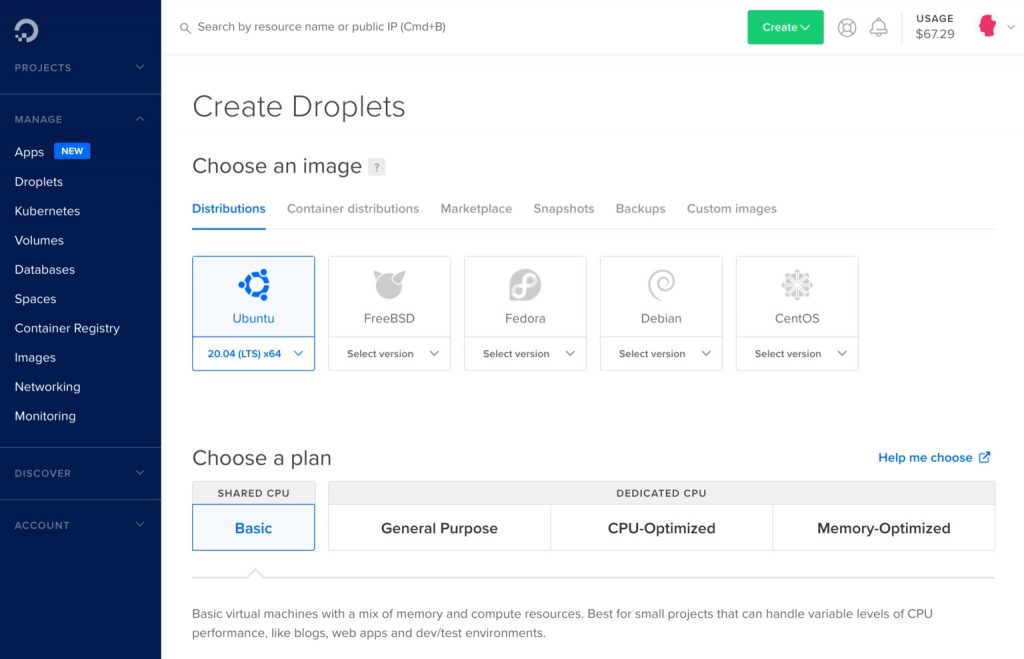Here's a cleaned-up and detailed caption:

"This desktop screenshot displays a management interface for a company's platform, likely related to cloud services or development projects. The primary menu is vertically aligned on the left side, featuring a blue section at the top emblazoned with the company's circular or 'O' shaped logo. Below this logo, the 'Projects' section is visible with a dropdown arrow. Expanding this menu reveals additional options: 'Manage' with an upward-pointing arrow to show further details, 'Apps' (highlighted as 'New'), 'Droplets', 'Kubernetes', 'Volumes', 'Databases', 'Spaces', 'Container Registry', 'Images', 'Networking', and 'Monitoring'. Further down, sections labeled 'Discover' and 'Account' each have dropdown arrows.

The main body of the interface features a search area at the top, alongside a 'Create' button with a dropdown arrow, various icons, and a financial summary for usage. Specifically, the 'Create Droplets' section allows users to choose an operating system image. Here, 'Ubuntu' is highlighted within a selectable box under the 'Distributions' tab. Directly beneath this, users have options to choose a plan, with 'Basic' currently selected."